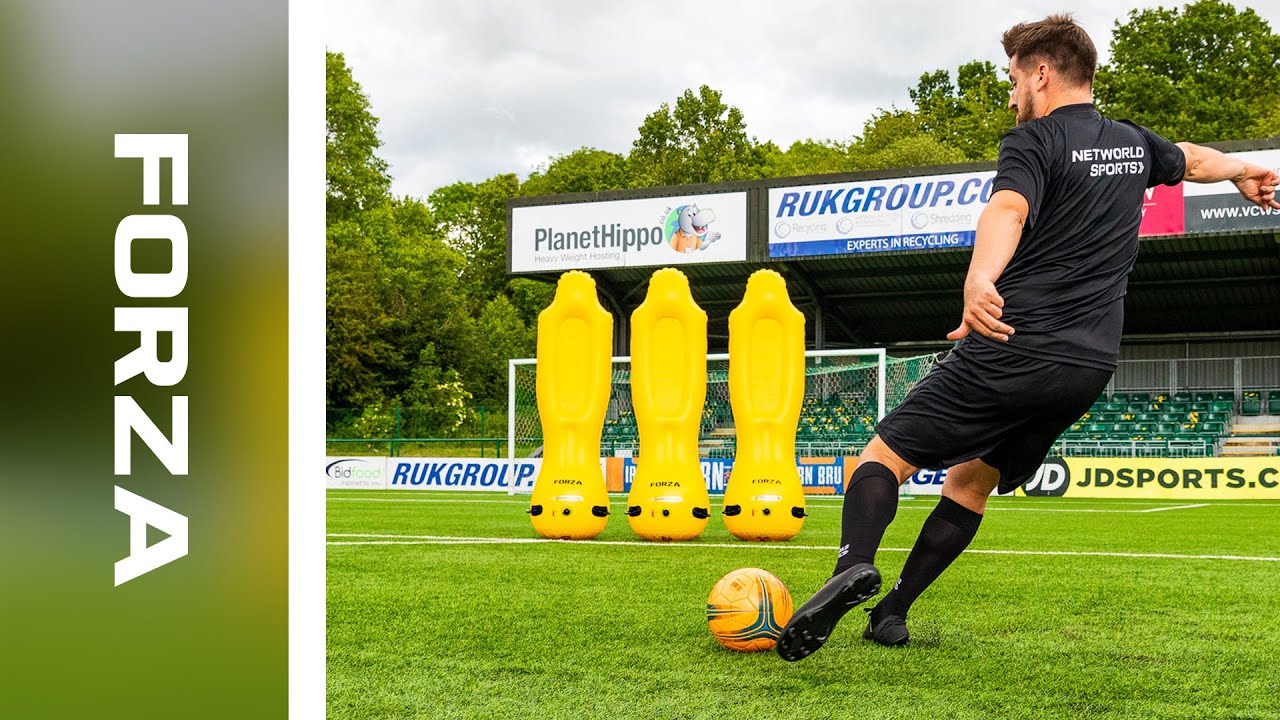In this detailed image, we see a man practicing soccer on a grassy field, presumably part of an advertisement for a sports company. The left side of the image features a blurred background with sideways white text that reads "FORZA." The main focus of the image is on the right side, where a man dressed entirely in black is about to kick a yellow soccer ball with black stripes using his left foot. He wears a short-sleeve t-shirt, shorts, knee-high socks, and soccer cleats, and the back of his shirt prominently displays the text "NET WORLD SPORTS" in white capital letters.

The man, who has short brown hair and facial hair, is running towards three yellow inflatable training dummies positioned in front of a soccer net. His arms are outstretched for balance, and he's in the act of executing what seems to be a penalty kick, aiming to curve the ball around the dummies.

Behind him, there is a small set of green stadium-style seats, largely empty, bordered by a white railing. Above these seats, various advertisements are visible, including ones for JD Sports, Planet Hippo, BidFood, and RUK Group. The setting appears to be in a partially forested area, adding a natural backdrop to the scene.